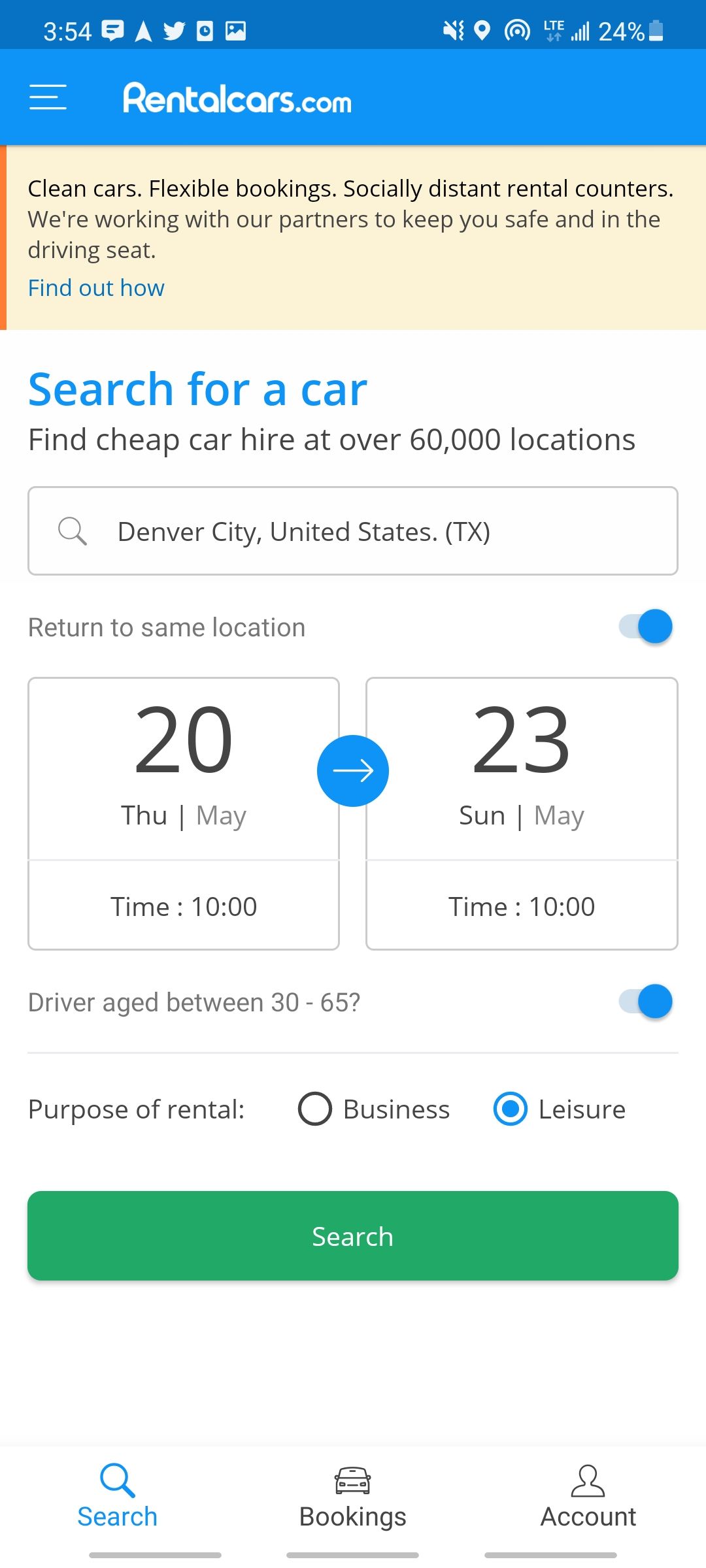The screenshot displays the Rentalcars.com app on a smartphone. The screenshot was captured at 3:54, as shown on the top left corner of the screen. The status bar indicates a strong Wi-Fi signal, LTE connectivity, the phone is set to vibrate, and the battery is at 24% charge.

At the top of the app, a yellow box highlights the message: "Clean cars, flexible booking, socially distant rental counters. We're working with our partners to keep you safe and in the driving seat, find out how." Below this message is the main interface where users can input their rental car preferences.

The search box under "Search for car" specifies: "Find cheap car hire at over 60,000 locations." The user has entered "Denver City, United States" in the state of Texas as their desired pickup location. An option is provided to return the car to the same location, which is currently toggled on. 

The user intends to rent the car from Thursday, May 20th to Sunday, May 23rd, with a specified rental time of 10:00 AM. There is a query about the renter's age, stating: "Age between 30 to 65?", with the toggle set to on. The purpose of the rental is also queried, with options for "business" or "leisure"; the "leisure" option is currently selected. 

At the bottom of the screen, there is a prominent green button labeled "Search," as well as navigation buttons for "Search," "Bookings," and "Account."